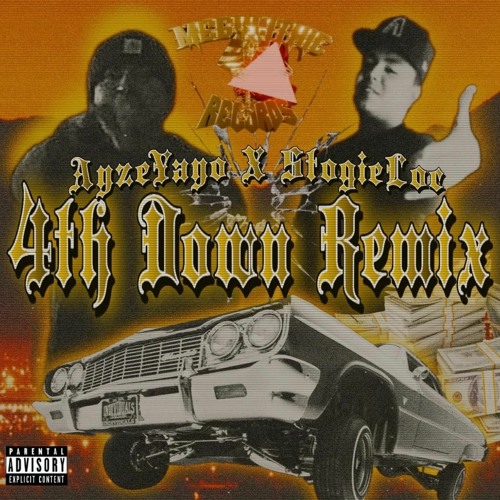This album cover features an orange sunset background with faint outlines of mountains and a nighttime cityscape at the bottom. Dominating the image are two black and white photos of two men, likely Hispanic rappers, positioned on the left and right. The man on the left wears a winter hat with a logo, while the man on the right sports a ball cap, possibly with a sports team logo, and is seen giving a thumbs-up.

Across the center, in a distinctive Gothic font, the text reads "Yangziyanga x Stokilor 4th Down Remix." Above this, in the very top middle, there's a part-hidden gold triangle that appears to represent the record label's name, which is partially obscured by a puppet holding a red triangle. Below the men, there is a black and white image of a car with hydraulics, depicting it mid-bounce with visible wheels and license plate. On the bottom right, bundles of money are scattered near the car. Finally, in the far bottom left corner, a "Parental Advisory: Explicit Content" label cautions about the graphic language within the album.